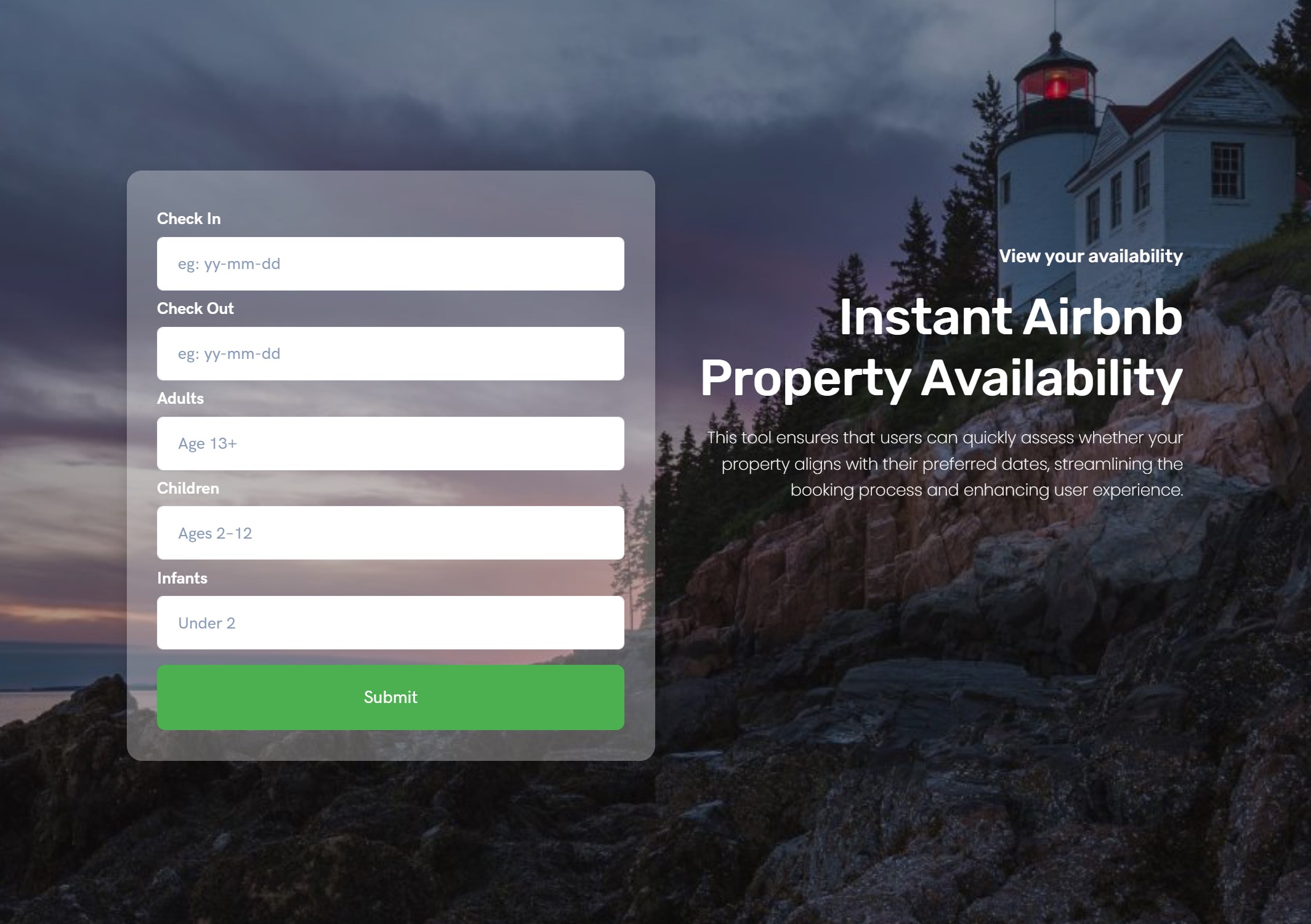This image is a screenshot of a webpage with a visually captivating background of a mountainside landscape, featuring a small, white lighthouse with a black roof located in the upper right corner. The lighthouse, which has a house attached to its base, stands out against the scenic backdrop.

Prominently displayed beneath the lighthouse, text in white font reads, "View your availability. Instant Airbnb property availability." This tool description further elaborates that it helps users quickly determine if their desired booking dates are available, thereby streamlining the booking process and enhancing the overall user experience. 

To the left of this descriptive text, there are five input fields, each bordered with a translucent gray outline and set against a white background for user entries. These fields are labeled as follows:

1. **Check-in:** This field prompts the user to enter the check-in date in the format "YYYY-MM-DD."
2. **Check-out:** This field prompts the user to enter the check-out date in the same format "YYYY-MM-DD."
3. **Adults:** This field is designated for specifying the number of adults aged 13 and above.

The interface appears clean, with the fields designed to be easily accessible and user-friendly, ensuring a smooth navigation experience.